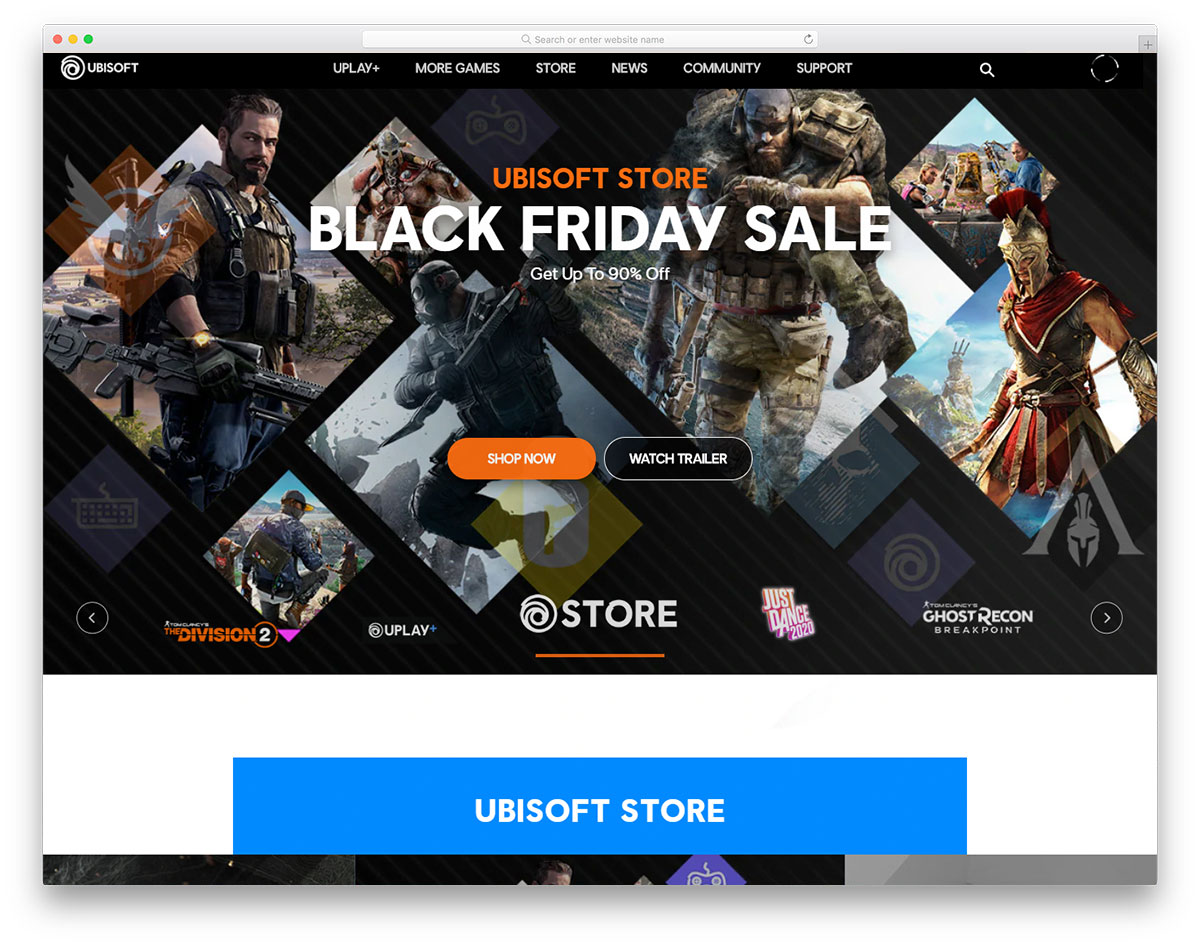The image is an advertisement from the Ubisoft Store, highlighting their Black Friday sale. The centerpiece prominently features the Ubisoft logo in vibrant orange text, and the announcement "Black Friday Sale" in bold white text, declaring discounts of up to 90% off. Surrounding this, the background showcases a montage of dramatic video game characters, including a notable warrior carrying another person over his back, emphasizing the company's array of action-packed games. At the bottom, there is a conspicuous "Shop Now" button in bright orange, accompanied by a "Watch Trailer" button in black. The screen is partially cut off, but it reveals a blue banner at the top with "Ubisoft Store" in all capital letters. Additionally, a navigation bar at the top offers tabs labeled "You Play," "More Games," "Store," "News," "Community," and "Support," providing various options for exploring the site further.